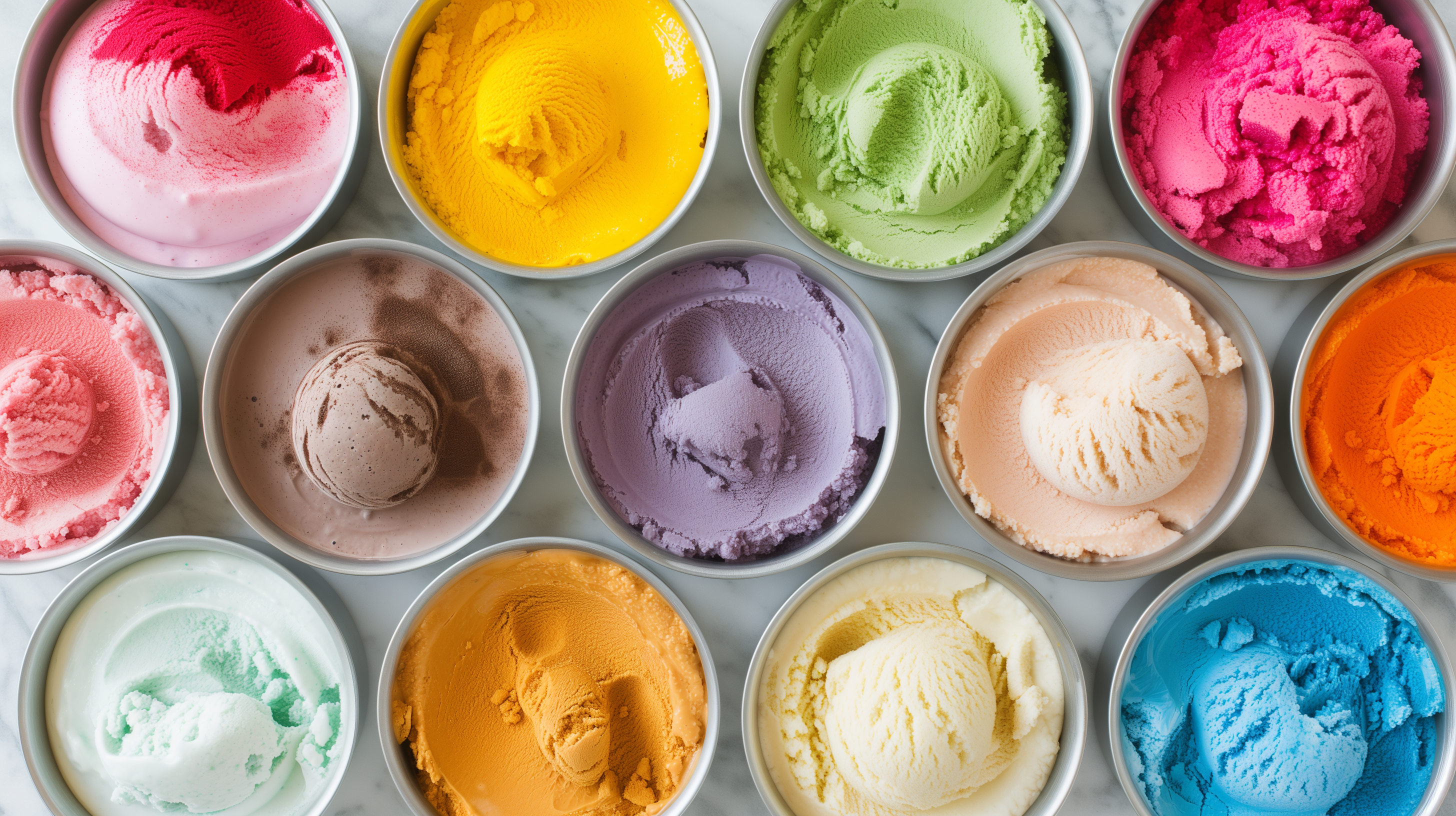This color photograph showcases an array of vividly colored ice creams in pint-sized containers, arranged in three neat rows on a white marble countertop and viewed from above. The top row features, from left to right, a light pink ice cream with a bright red swirl, a yellow ice cream, a mint green ice cream, and a bright pink ice cream. The middle row includes a darker pink ice cream, a brown ice cream, a lavender ice cream, a light orange ice cream, and a deep orange ice cream. The bottom row displays a light blue ice cream, a golden butterscotch ice cream, a classic white vanilla ice cream, and a pastel blue ice cream. The lids are removed to reveal the rich, colorful textures, with scoops taken out of the middle of each carton, highlighting the array of flavors.